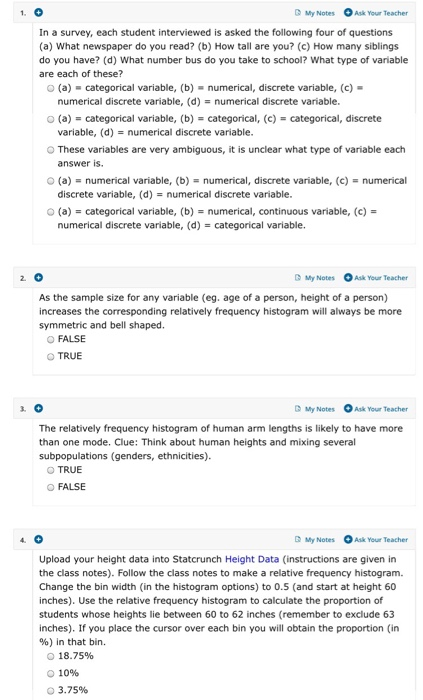### Detailed Caption:

This image is a screenshot of a digital educational webpage displaying a set of four survey questions aimed at students. The content is written in black font on a standard-size display with minimal variation in formatting. Positioned at the top right-hand corner of the page are two interactive options labeled "My Notes" and "Ask Your Teacher," allowing students to either refer to their notes or seek assistance from their teacher.

Below this header, the page is organized into a structured questionnaire. The survey questions are numbered sequentially from 1 to 4 down the left-hand side of the page. 

1. **Question 1:** This is a multi-part question where each student is asked:
   - **A.** Which newspaper do you read?
   - **B.** How tall are you?
   - **C.** How many siblings do you have?
   - **D.** What number bus do you take to school?
   The task for students is to identify the type of variable for each of these sub-questions. Five options are provided to choose from.

2. **Question 2:** A concise true-or-false question.

3. **Question 3:** Another brief true-or-false question.

4. **Question 4:** This question presents three different answer options in the form of percentages.

The entire content appears to be formatted for academic purposes, possibly aimed at students studying survey methodology or statistical analysis.